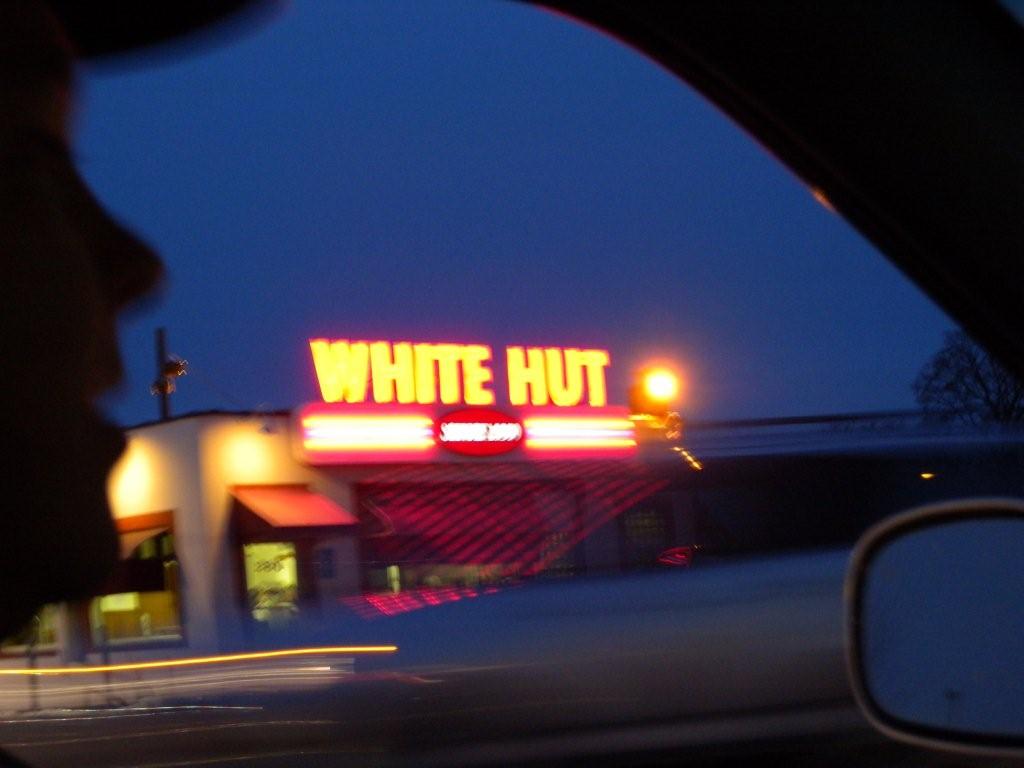The image presents a driver's perspective from inside a car, looking out onto a restaurant named "White Hut." In the top left corner, the driver's face is partly visible from a side angle. The bottom right corner features the car’s side mirror, which has a gray outer frame and a light gray interior reflecting the surroundings. The scene outside includes a gray road and a gray parking lot with a yellow horizontal light illuminating the area. Dominating the view is the restaurant building itself, also gray, with a sign reading "White Hut" in yellow letters prominently displayed at the top. Just below this sign is a red, oval-shaped sign with white text. Additional lights flank the restaurant on both sides. The car’s black frame is seen in the top right corner of the image, and a clear blue sky forms the backdrop above the restaurant.